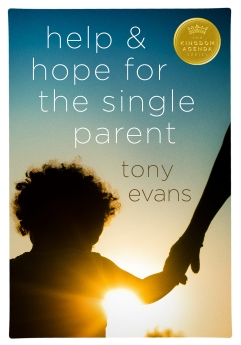The cover of the book, "help and hope for the single parent" by Tony Evans, features a poignant image and thoughtful design that encapsulate its inspirational theme. The title is prominently displayed in lowercase white letters at the top of the cover. Tony Evans' name appears just below it in a warm beige or orangish color. In the upper right corner, a gold seal with a crown and the inscription "the kingdom agenda" lends a regal touch to the design.

The cover image is strikingly symbolic: Against a gradient background that transitions from dark blue at the top to light blue at the bottom, a child with curly hair, depicted as a silhouette, stands in the lower left corner. The child's right hand reaches up to hold the left hand of an adult, who is partially visible, also as a shadow. Sunlight shines through beneath the child's right armpit, casting a hopeful glow across the scene. At the very bottom, the tips of tree branches or a bush can be seen, also illuminated by the sun's rays. This imagery of a guiding hand leading a child towards sunlight visually reinforces the book's message of support and optimism for single parents.